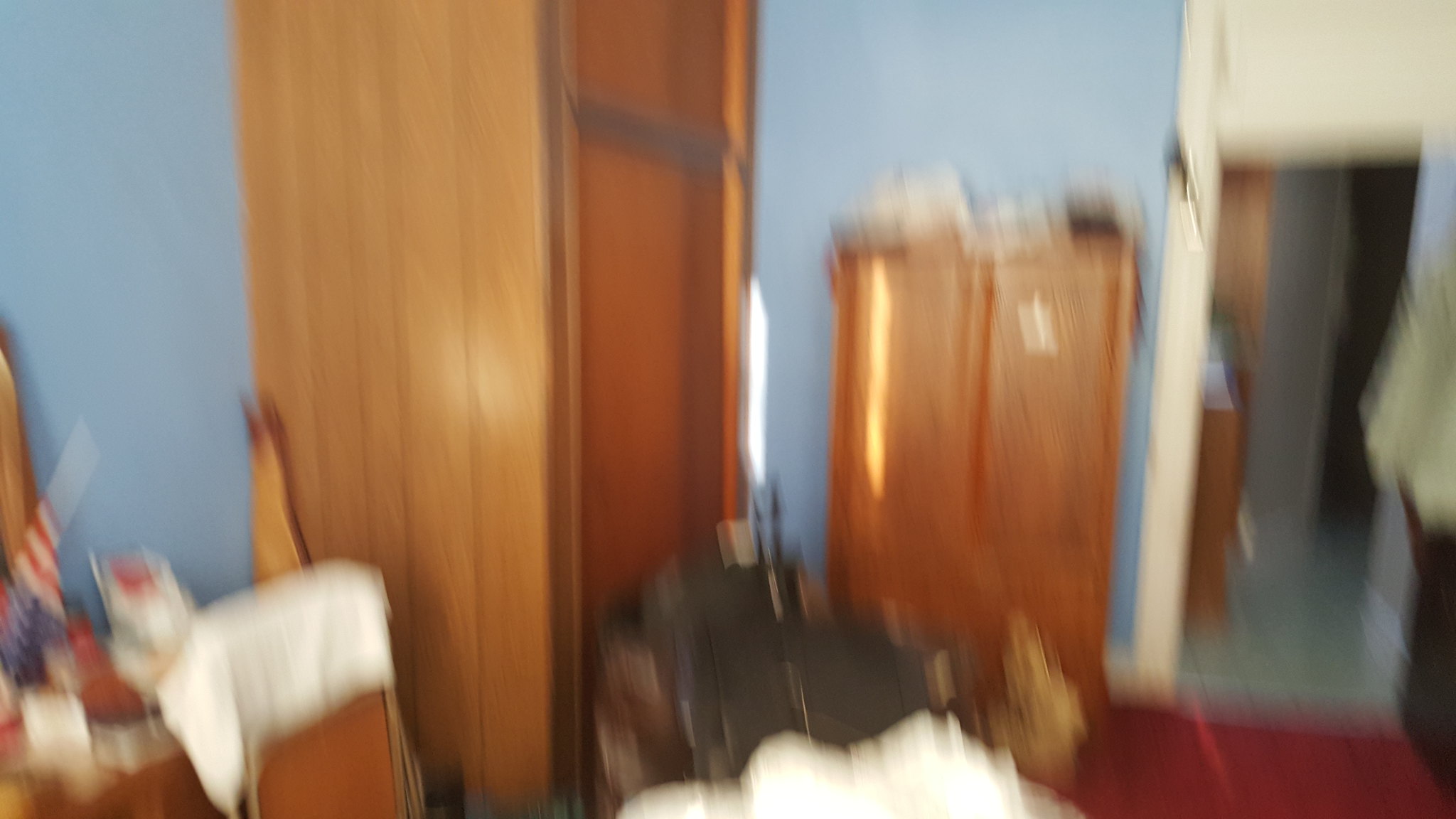The image is a very blurry photograph of a room, most likely a bedroom, with light blue walls and white trim. The camera appears to have been moved while the picture was taken, adding to the difficulty of discerning details. The floor is a reddish maroon color. In the foreground, on the bottom right, there's part of a chair with a white towel draped over it and what appears to be a small American flag upside down, possibly on a desk or vanity. Straight ahead, we see two large honey brown pieces of wooden furniture that seem to be an armoire or dresser and a coat closet. The piece to the right is just a bit shorter than a nearby hallway doorway, which leads to a darker area with blue and gray tones, possibly a kitchen or bathroom indicated by what looks like a tiled floor. In the background, there are some white and black objects on top of the furniture and a mirror on a white wall. The image also includes several indiscernible items due to the blurriness, including a possible black suitcase and more clutter in the middle bottom of the picture.